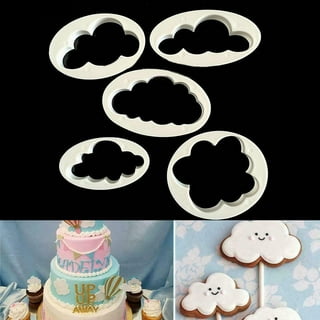The image consists of three small sections that collectively present a detailed scene of cake decorating. The top section showcases five cloud-shaped cookie cutters arranged against a black background. The bottom left section features a multi-layered cake decorated elaborately: the bottom tier is white and features the text "Up, Up, Away" with a drawing of a hot air balloon to its right. The middle tier is blue with cloud decorations, while the top tier is pink and adorned with a banner. Surrounding the cake are several cupcakes, complementing the theme. The bottom right section displays cookies in the shape of fluffy clouds, some of which have little smiley faces. These cloud cookies are mounted on white wooden pegs and set against a blue flowered background.